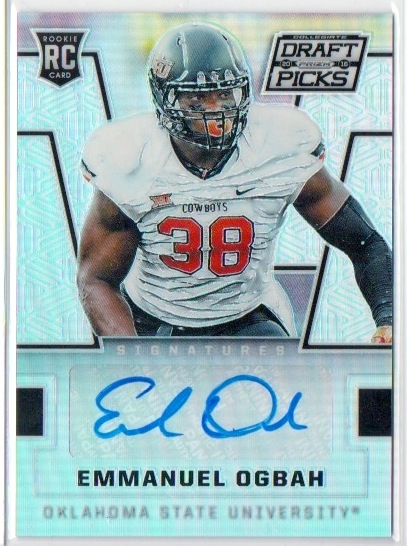This rectangular trading card features a dynamic image of a football player mid-run during a game. The player, wearing a black helmet, eye paint, and an orange mouth guard, is dressed in a white jersey emblazoned with "Cowboys" and the number 38 in bold red. His left arm is covered with a black sleeve. The top left corner of the card displays a badge labeled "Rookie RC Card," while the upper right corner features a logo that reads "Draft Picks" in black text on a gray background. Below the player's waist, where the image cuts off, is a box labeled "Signatures" containing his autograph in blue ink. The printed name "Emmanuel Ogbah," spelled O-G-B-A-H, is situated below the signature, followed by "Oklahoma State University." The card's background sports a faded turquoise hue with various patterns, including a cross-hatched design behind the player and a simpler, plainer pattern in the lower section.